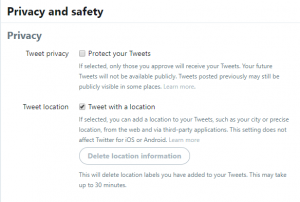The image displays a section from a social media platform, specifically Twitter's "Privacy and Safety" settings. It shows options related to "Privacy" and "Tweet Privacy." The section outlines features such as "Protect your Tweets," indicating that if this option is selected, only approved followers will receive your tweets, and future tweets will not be publicly available. Previously posted tweets may still be visible publicly in some areas, with a "Learn more" link provided for additional information.

Another feature shown is "Tweet location," which explains that if selected, users can add a location to their tweets, such as their city or specific location, via the web and third-party applications. It notes that this setting does not apply to the Twitter app for iOS or Android, with another "Learn more" link available for further details.

Additionally, the image highlights the "Delete location information" option, which allows users to delete location labels previously added to their tweets. A note mentions that this process may take up to 30 minutes. In the image, this particular option is already selected.